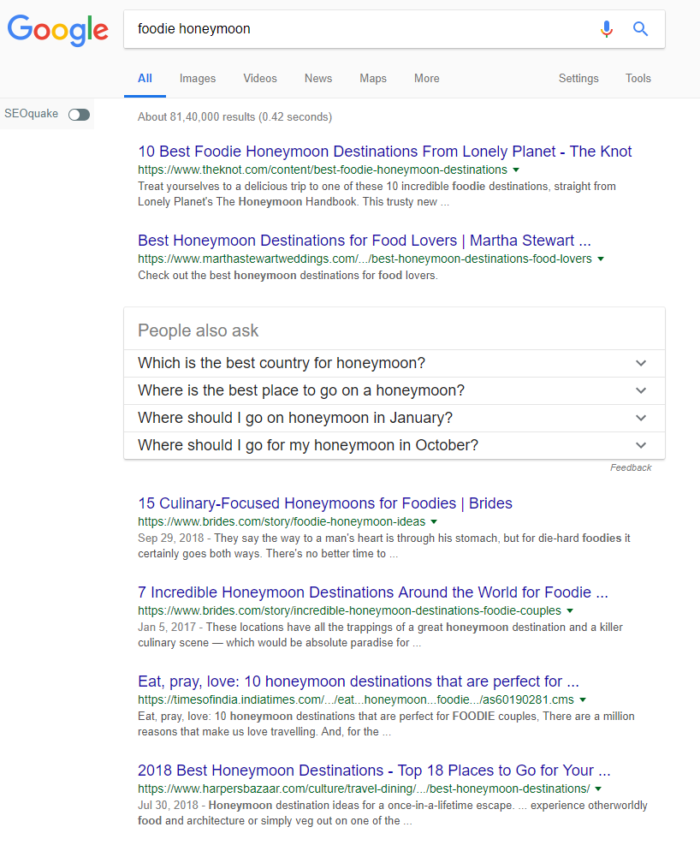The image displays a Google search page in day mode, characterized by its white background. In the upper left corner, the Google logo is prominently visible. The search query entered in the search bar reads "foodie honeymoon" in lowercase letters. Adjacent to the search bar on the right are a microphone icon and a blue search icon.

Directly below the search bar are various search filter tabs, with "All" selected, highlighted in blue and underlined. Following tabs include "Images," "Videos," "News," "Maps," and "More." Further to the right, options for "Settings" and "Tools" are visible.

Below these tabs, on the left, there is a mention of "SEO Quake," a browser extension that is currently disabled, indicated by a gray slider. To the right, in gray text, are the search results statistics, showing approximately 81,400,000 results found in 0.42 seconds.

The search results begin with the first blue or purple headline which reads, "10 Best Foodie Honeymoon Destinations from Lonely Planet, The Knot." The URL is displayed in green as "https://www.thenot.com/content/best-foodie-honeymoon-destinations," followed by a brief description about a delicious trip to top foodie destinations, which is cut off towards the end.

The second result is titled "Best Honeymoon Destinations for Food Lovers," credited to Martha Stewart, with the URL "marthastewartweddings.com." It encourages readers to explore the best honeymoon destinations for food enthusiasts.

Below these top search results, a box titled "People also ask" features frequently asked questions related to honeymoons. Questions include:
- "Which is the best country for honeymoon?" with an expandable arrow on the right.
- "Where is the best place to go on a honeymoon?" with a similar arrow.
- "Where should I go on honeymoon in January?" also with an arrow.
- "Where should I go for my honeymoon in October?" again, with an arrow. Beneath these questions, a "Feedback" link is visible in gray text.

Further down, additional search results are displayed including:
- "15 Culinary Focused Honeymoon Foodies by Brides," listed on brides.com from September 29, 2018.
- "7 Incredible Honeymoon Destinations Around The World For Foodies," also from brides.com, dated January 5, 2017.
- "Eat, Pray, Love: 10 Honeymoon Destinations That Are Perfect For Foodie Couples" from The Times of India, with the URL "indiatimes.com."
- "2018 Best Honeymoon Destinations: Top 18 Places to Go For Your," listing partially cut off from www.harpersbazaar.com, dated July 30, 2018.

This detailed view emphasizes the variety of information delivered by the search, reflecting a wide array of content aimed at couples seeking the best foodie honeymoon experiences.